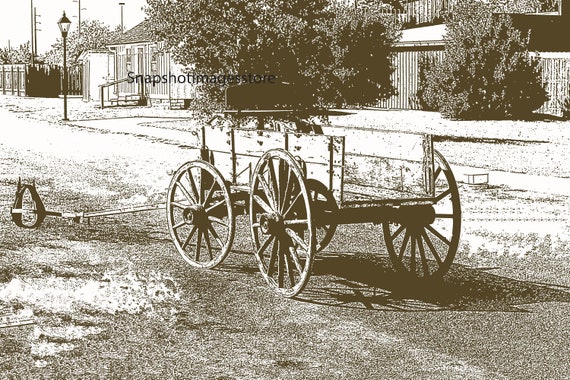This black-and-white image appears to be a vintage photograph of an urban street scene. Central to the composition is an empty, U-shaped wooden buggy, indicative of a horse-drawn vehicle, positioned directly in the middle facing forward along a muddy dirt road. Surrounding the buggy, we see several period-appropriate details: a lamppost situated in the top left corner, streetlights, and power poles scattered throughout the scene evoking an old-town ambiance. Buildings frame the middle top and right corners, with bushes nestled in front of them, adding to the nostalgic feel. There is a distinct watermark across the front of the buggy that reads "Snapshot Mag Store." Despite its antique appearance, some speculate the photograph might be modern with a sepia-toned filter, given the clarity and presence of contemporary details. This image captures a serene yet bustling urban setting and might date back to anywhere from the 1910s to the 1940s.